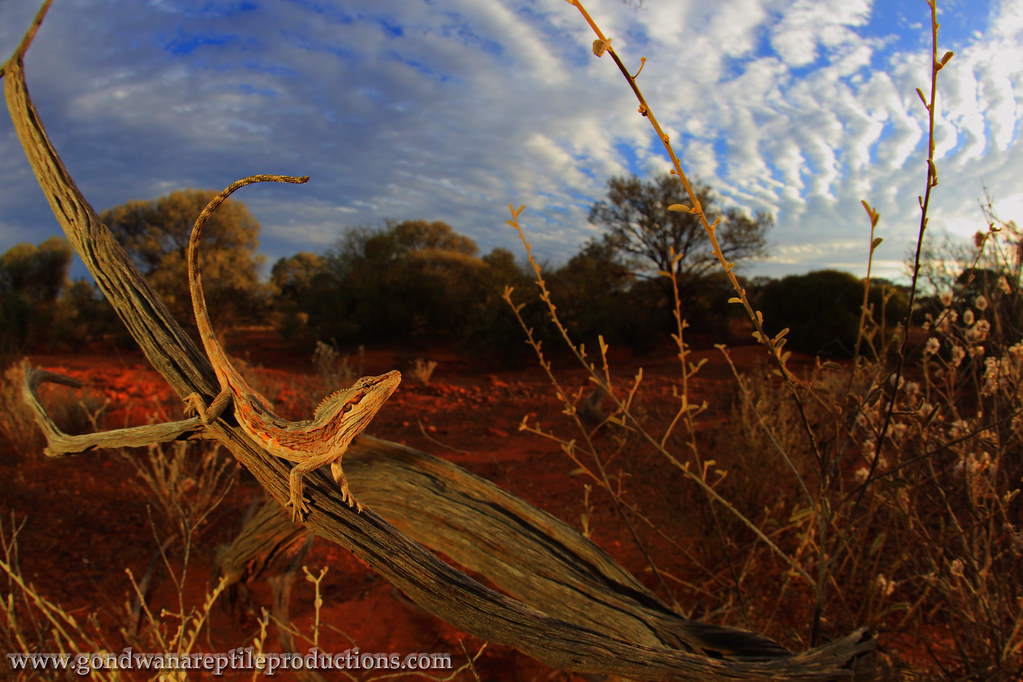The photograph captures a desert terrain featuring a detailed scene with prominent natural elements and vivid colors. In the foreground, a lizard, primarily gray with hints of orange, stands alert on a dead, brown branch situated towards the middle-left of the image. The lizard has its head and tail raised, giving it a dynamic posture. To the right of the branch, dried-out brush and tumbleweeds with petite florals are visible, adding texture to the arid landscape. The background displays darkened trees, likely shaded by the positioning of the sun. The sky above is a striking blue adorned with white, rippled clouds. Whites, blues, browns, greens, and reddish tones dominate the color palette, creating a vibrant yet earthy atmosphere. In the bottom-left corner, white text reads "www.gond1r1anareptileproductions.com," indicating the source of this reptile-centric image, likely from their website dedicated to various reptiles, including lizards and potentially snakes.